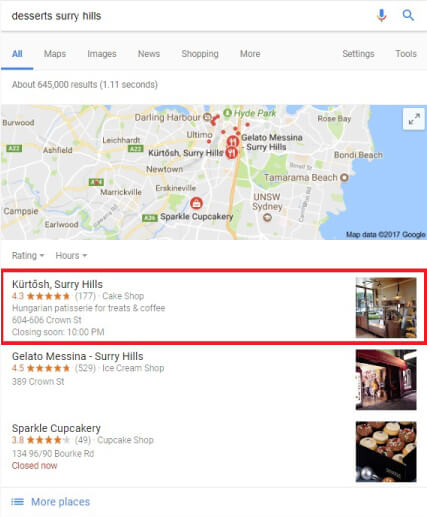Detailed caption: 

This image depicts a search results page for "desert Surrey Hills" on Google, with the key elements highlighted in blue. The interface includes options such as maps, images, news, shopping, as well as settings and tools. A detailed map showcasing various cities surrounding the Surrey Hills area is prominently displayed. Below the map, specific search results are featured, starting with Kirtosh Surrey Hills, a Hungarian pastry shop located on Crown Street. This shop, known for its treats and coffee, has a 4.3-star rating and is noted to be closing soon at 10 PM. 

Further down, Gelato Messina Surrey Hills is highlighted, boasting a noteworthy five-star rating and specializing in ice cream. Sparkle Cupcakery, another featured shop, is a cupcake establishment with a four-star rating and is currently closed. Accompanying these text results are various images depicting the shops and their offerings: Sparkle Cupcakery showcases a selection of beautifully decorated cupcakes, while Gelato Messina is represented by a slightly obscured shot of the ice cream shop with two people entering. Kirtosh Surrey Hills is seen in an image taken during the daytime, offering an interior view of the pastry shop. The map data is sourced from Google and dates back to 2017.